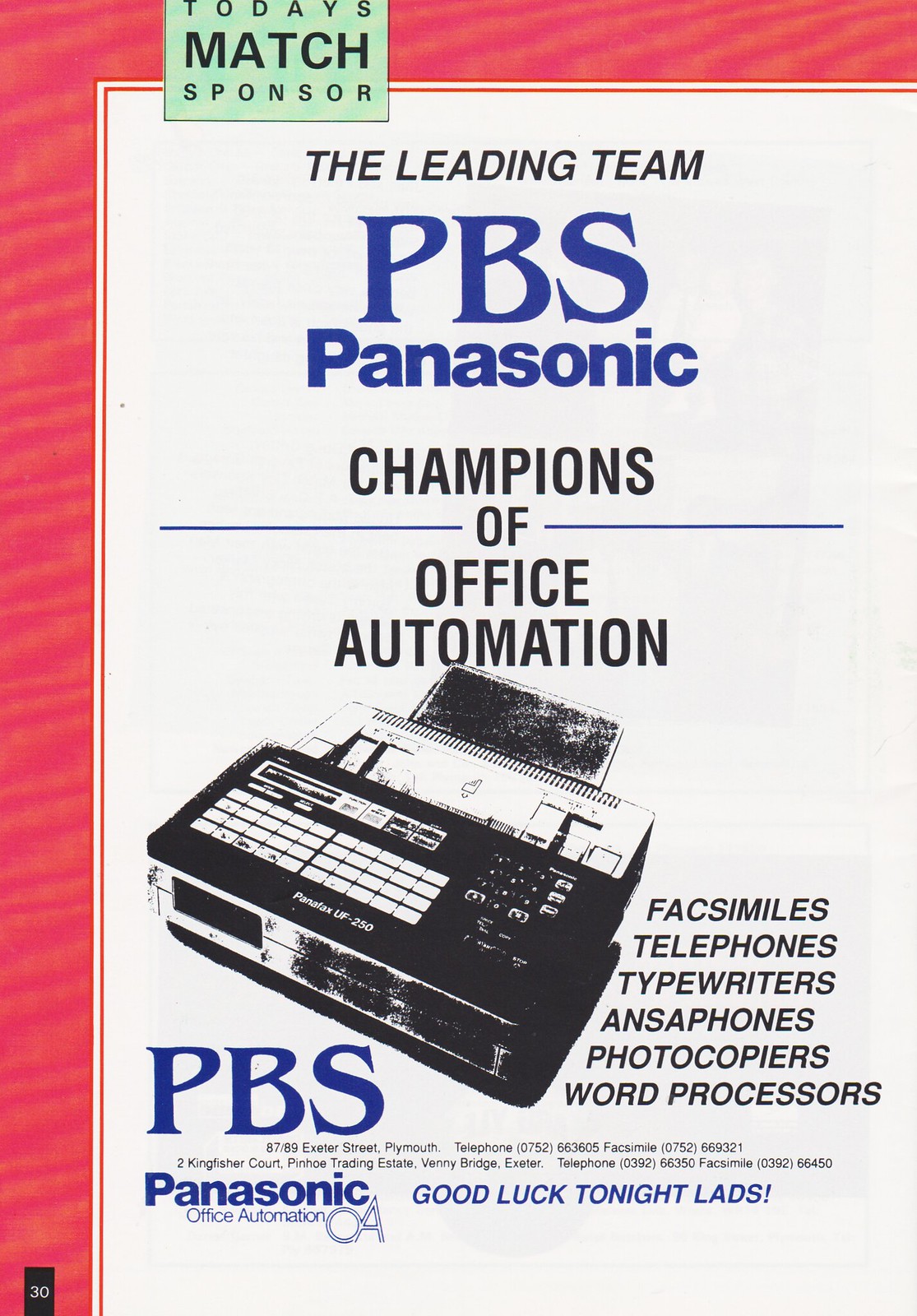This image is a detailed sponsor advertisement from a vintage football club program. It features a prominent Panasonic brochure, characterized by a distinctive red border along the left edge and top bar. The page, printed in black and white with selective use of red and blue highlights, is marked as page 30 in the program. At the top, a green text box with black text announces "Today's Match Sponsor," intersected by a red horizontal and vertical stripe.

Beneath this, the title "The Leading Team" appears in bold black text, followed by "PBS Panasonic" in larger, dark blue font, firmly establishing brand presence in the top third of the image. The tagline "Champions of Office Automation" is centered below the title. 

The lower third of the page showcases a black-and-white image of a Panasonic fax machine, accompanied by a neatly aligned list of office products to the right: "Facsimiles, Telephones, Typewriters, Answer Phones, Photocopiers, Word Processors." Towards the bottom, a message reads "Good luck tonight lads!" with the PBS logo situated in the bottom left corner. The overall style is reminiscent of a vintage print publication, effectively blending textual information with illustrative elements.